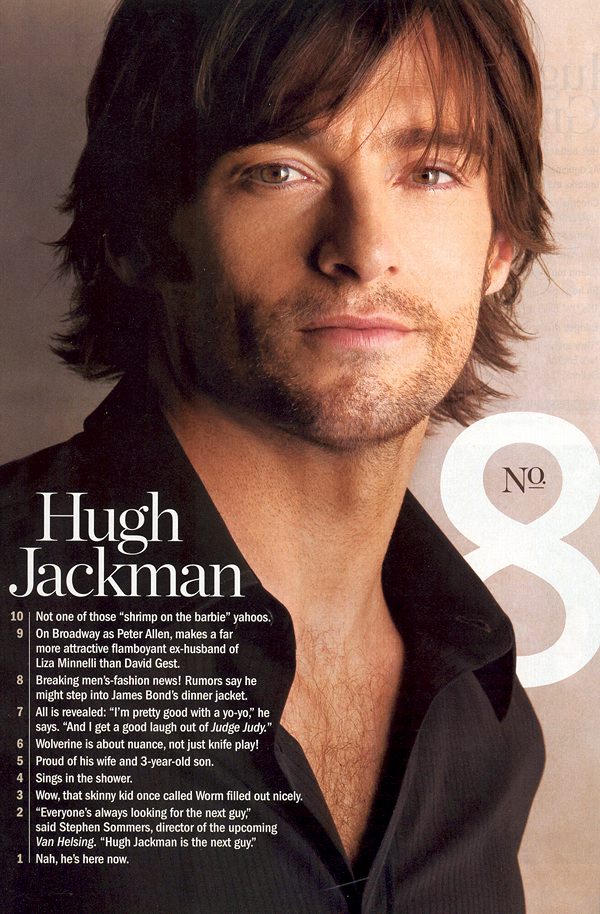This promotional poster features a young Hugh Jackman, showcasing his tousled, layered dark brown hair and a slightly unshaven look with a bit of a mustache and beard. He's facing forward, directly gazing at the camera, giving the impression of confidence. Jackman is donning an open black collared shirt with the top two or three buttons undone, revealing a hint of chest hair. The background is a light-colored wall.

Prominently displayed on his right shoulder, in large white letters, is his name: "Hugh" above "Jackman." Below his name, there are approximately 15-17 lines of white text spanning across his right chest and shoulder. To the left of these lines are numbers, starting at 10 at the top and descending to 1 at the bottom.

Highlighted within the text are certain notable points: 

- "Hugh Jackman, not one of those shrimp on the barbie yahoos."
- "On Broadway as Peter Allen, makes a far more attractive flamboyant ex-husband of Liza Minnelli than David Jest."
- "Breaking men's fashion news, rumors say he may step into James Bond's dinner jacket."

The numbers form a countdown, emphasizing Jackman's significance, concluding with a line at 1 that states, "Nah, he's here now."

This detailed and structured layout effectively captures and promotes Hugh Jackman's charismatic and versatile image, further establishing his presence in both the film and fashion industries.